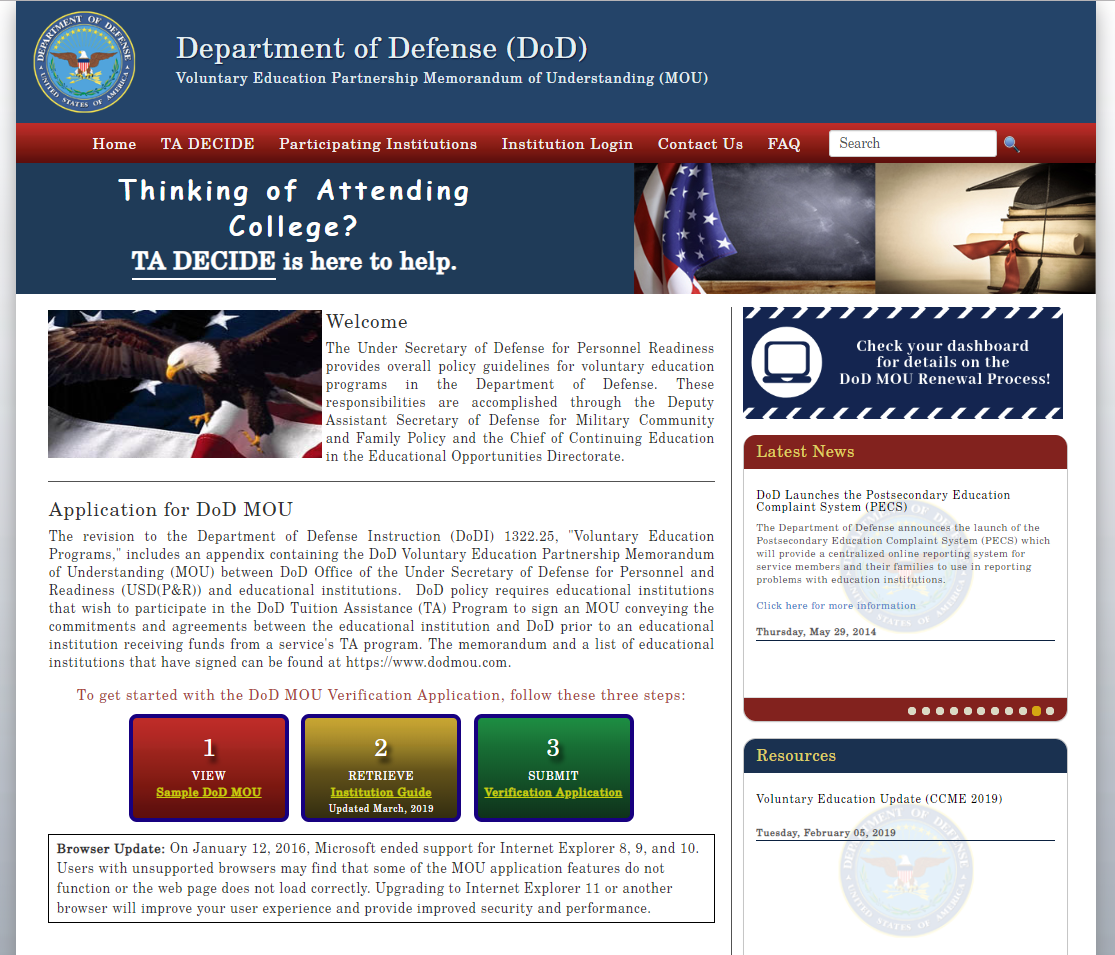The image appears to be a detailed screenshot of the official Department of Defense web page dedicated to the Voluntary Education Partnership Memorandum of Understanding (MOU). At the top, a blue navigation bar prominently displays the title "Department of Defense Voluntary Education Partnership Memorandum of Understanding (MOU)". On the left side, there is a distinguished seal featuring an eagle and encircling text that reads “Department of Defense”. Beneath this, a red navigation bar contains various links labeled "Home," "TA DECIDE," "Participating Institutions," "Institution Login," "Contact Us," and "FAQ." To the right of this navigation bar is a search bar, accompanied by a prompt that reads, "Thinking of attending college? TA DECIDE is here to help."

The main section of the page showcases two stock images side by side: one depicts an American flag next to a black chalkboard, while the other displays a stack of books topped with a graduation cap. Below these images, a white section contains text that offers a warm welcome and informs visitors about the role of the Undersecretary of Defense for Personnel Readiness in providing policy guidelines for voluntary education programs within the Department of Defense. The responsibilities are carried out through the Deputy Assistant Secretary of Defense for Military Community and Family Policy and the Chief of Continuing Education in the Educational Opportunities Directorate.

Additionally, the text explains the application process for the DOD MOU, referencing a revision to the Department of Defense Instruction (DODI) 132.25 regarding voluntary education programs. This revision includes an appendix detailing the DOD Voluntary Education Partnership Memorandum of Understanding (MOU) between the DOD Office of the Undersecretary of Defense for Personnel and Readiness (USD(P&R)) and educational institutions.